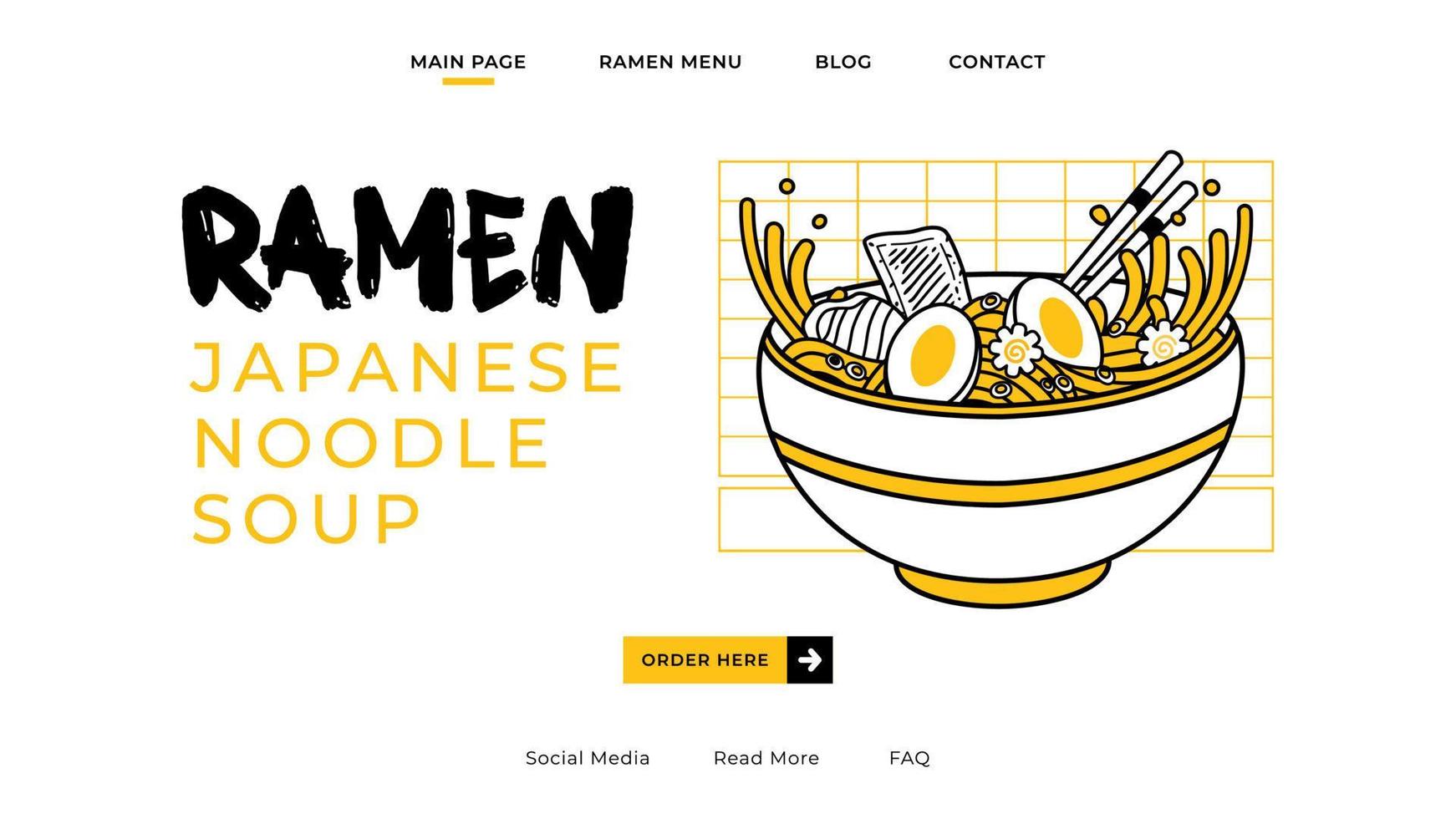The image depicts the main page of a website, likely for a restaurant specializing in ramen. The background is white with contrasting black text. Dominating the visual is an illustrative and stylized golden orange-yellow bowl of ramen located on the left. The bowl is detailed with black outlines, a single orange stripe along its body, and an orange base, filled with illustrated orange noodles, egg halves, circles, and flower shapes. Chopsticks are poised in the bowl as well. Adjacent to this illustration on the right, bold black text spells out "RAMEN" with smaller text underneath that reads "Japanese Noodle Soup."

In the center of the page, there's an orange rectangle featuring the text "Order Here" in black, coupled with a white arrow in a black square pointing to the right. At the bottom, horizontal black text provides navigation options labeled as "Social Media," "Read More," and "FAQ."

The top navigation bar includes four menu options: "MAIN PAGE" with a small yellow bar underneath, "RAMEN MENU," "BLOG," and "CONTACT," all written in capital letters.